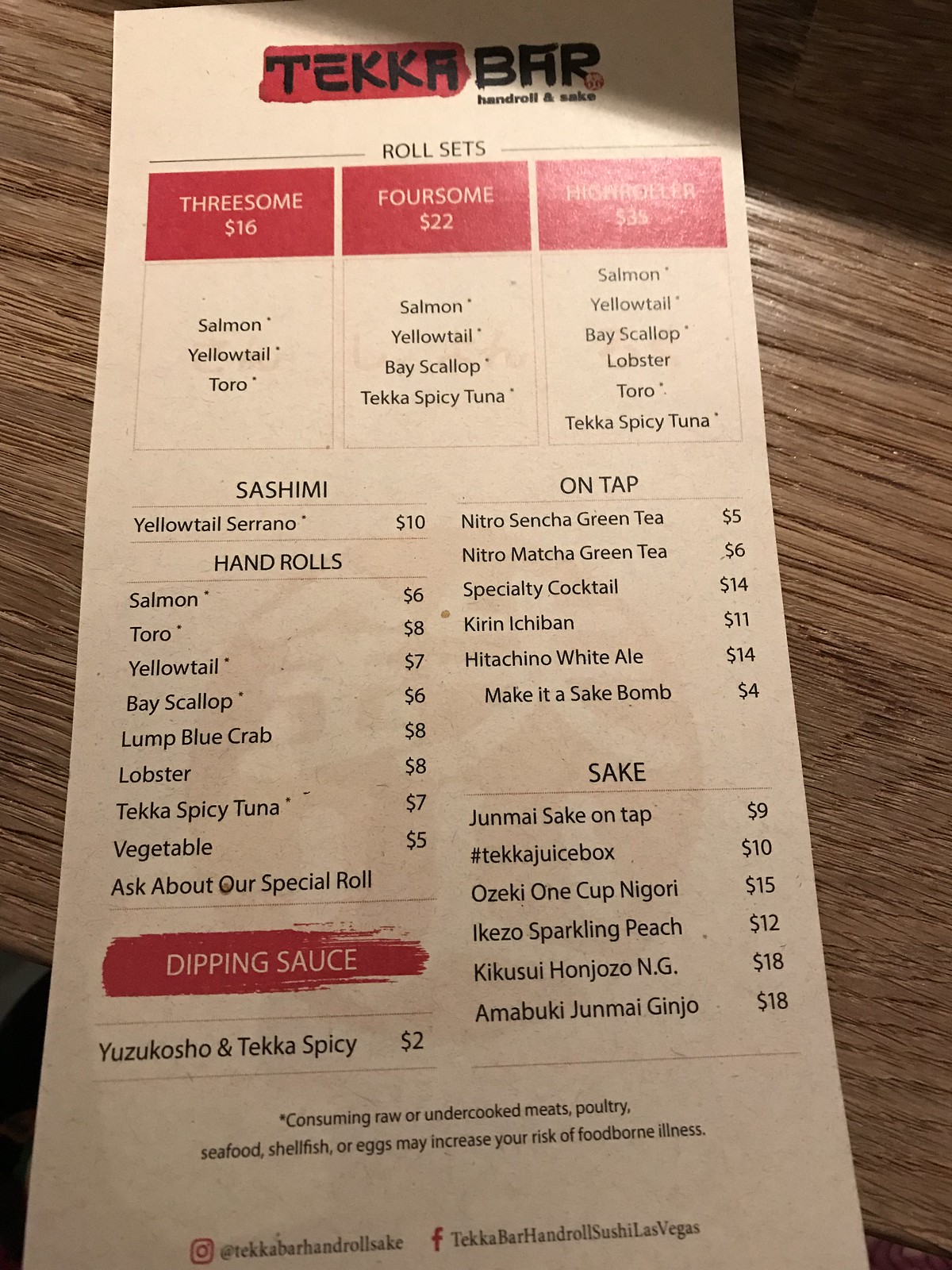This vibrant color photograph showcases a beautifully set menu on a blonde hardwood table. The menu, which dominates the frame, is elongated and printed on a very pale pink paper. The top of the menu features the logo of the establishment, "Teka Bar" (spelled T-E-K-A), presented in a distinctive style with "Teka" in black against a red oblong background.

Beneath the logo, the header "Roll Sets" appears, followed by three red squares with white text detailing set prices: "threesome, $16" and "foursome, $22." Unfortunately, the third option is obscured by glare. Beneath the threesome and foursome options, partially legible text suggests ingredients like salmon, reinforcing the menu's sushi-focused offerings.

The menu is divided into sections: on the left, a column lists various sushi options under headings like "sashimi" and "hand rolls," featuring ingredients such as salmon, bay scallop, lobster, and vegetable. On the right, another column outlines drink offerings under headings like "on tap" and "sake," listing beverages such as specialty cocktails, nitro matcha green tea, and multiple types of sake, appealing to a wide range of tastes.

Overall, the clean, organized layout of the menu, combined with the elegant hardwood table background, suggests a sophisticated yet inviting dining experience at Teka Bar.